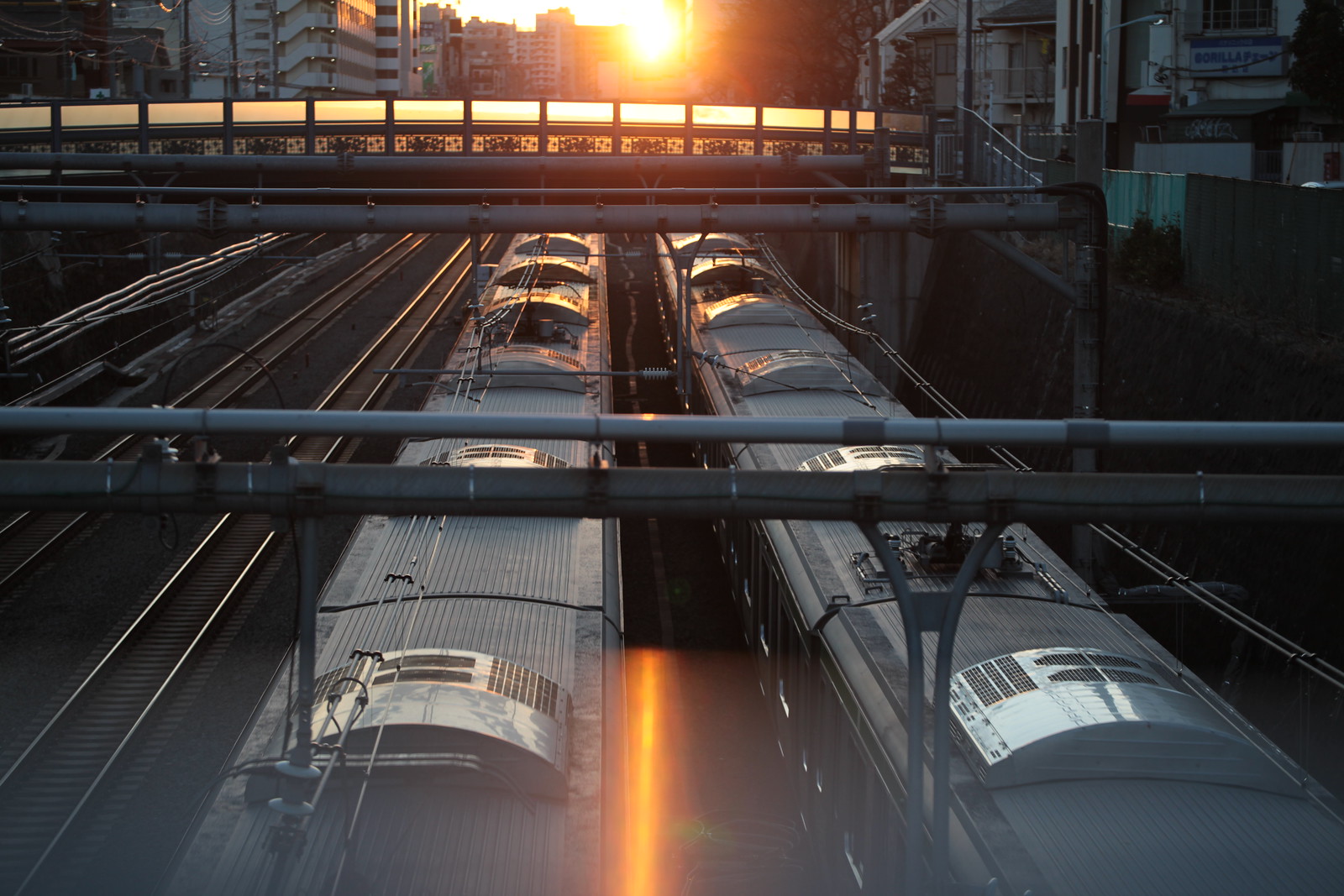This detailed photograph captures a top-down, landscape-oriented view of a vibrant cityscape at sunset. Four parallel railroad tracks run beneath a pedestrian bridge, and two gleaming gray metal passenger trains, resembling typical subway cars with fan vents on top, are seen traveling side by side towards the orangey glow of the setting sun. The sun, almost touching the horizon, bathes the scene in a warm, radiant light that highlights the bustling commercial buildings and the older neighborhood to the right. Metal pipes, wires, and the concrete surroundings frame this urban tableau, while the street above the trains and the distant city skyline add to the complexity and allure of this metropolitan landscape.